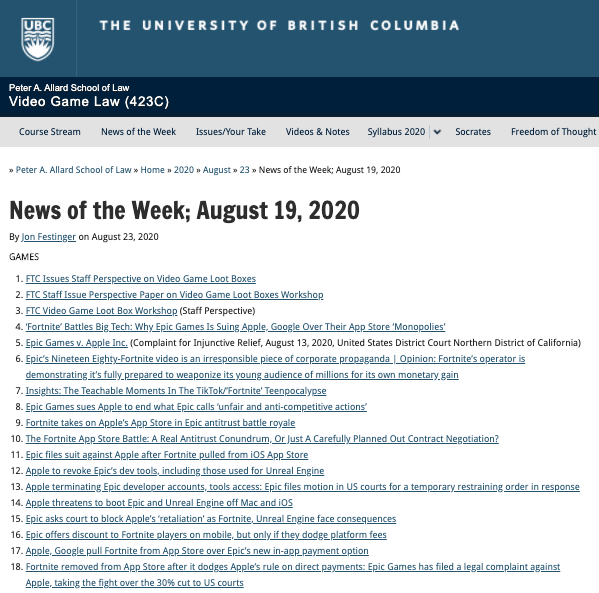This screenshot captures a webpage from the University of British Columbia, specifically the Peter A. Allard School of Law's section on Video Game Law (marked 4, 2, 3, C). In the top left corner, the university's shield is prominently displayed; the shield features the letters "UBC" in white, above a white-outline palm leaf design with three wavy lines situated between the letters and the palm frond.

The page highlights an article titled "News of the Week, August 19, 2020," authored by John Festinger and published on August 23, 2020. The article is centered on legal news and developments pertaining to video games. Below the article's header, there is a comprehensive list of 18 news items, each numbered in black and accompanied by hyperlinks to detailed news stories. For instance, the first item reads, "FTC Issues Staff Perspective on Video Game Loot Boxes."